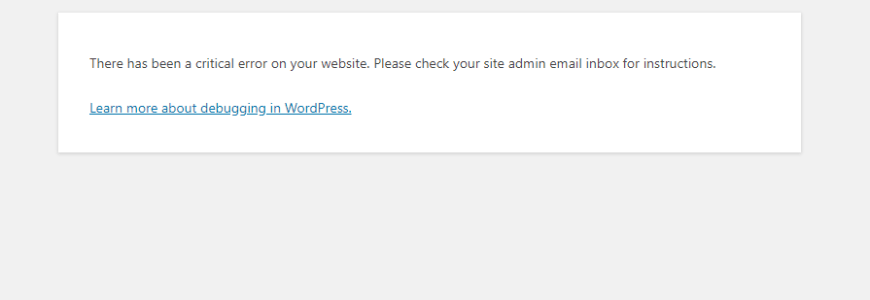In the image, a critical error message is prominently displayed against a white rectangular background. The main text, written in light black color, reads, "There has been a critical error on your website. Please check your site admin email inbox for instructions." Below this text, there is a hyperlink in blue that states, "Learn more about debugging in WordPress." The white rectangular background is set against a light gray backdrop, offering clear contrast to the messages. The image is rectangular in shape, being significantly wider than it is tall.